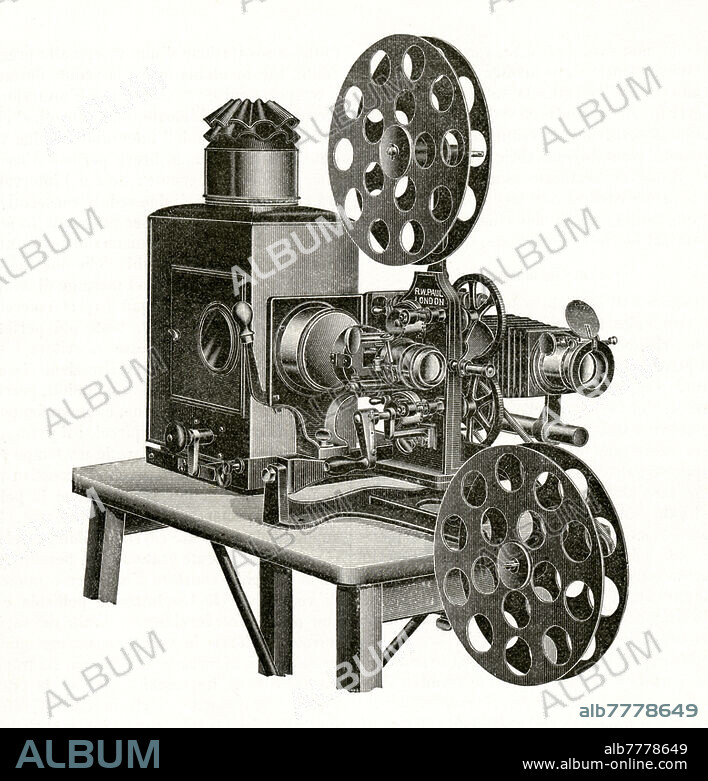This black and white line drawing depicts a vintage film projector, possibly from the early 1900s, identified as an antique Bodo projector or an early movie camera by RW Paul London. The intricately detailed apparatus features two large film reels—one for loading the film and another for take-up—along with multiple lenses, dials, gears, and a crank. It is securely positioned on a wooden table with visible legs, and a sizable box-like structure is attached to the back, possibly serving as a housing or chimney. The entire image is watermarked diagonally with the word "Album" in white embossed text, and additional branding is present at the bottom. Here, a black banner displays the text "Album" in blue-gray, alongside the code "ALB7778649" and the URL "www.album-online.com." This consistent watermarking and text suggest the image is a stock photo from the Album collection.